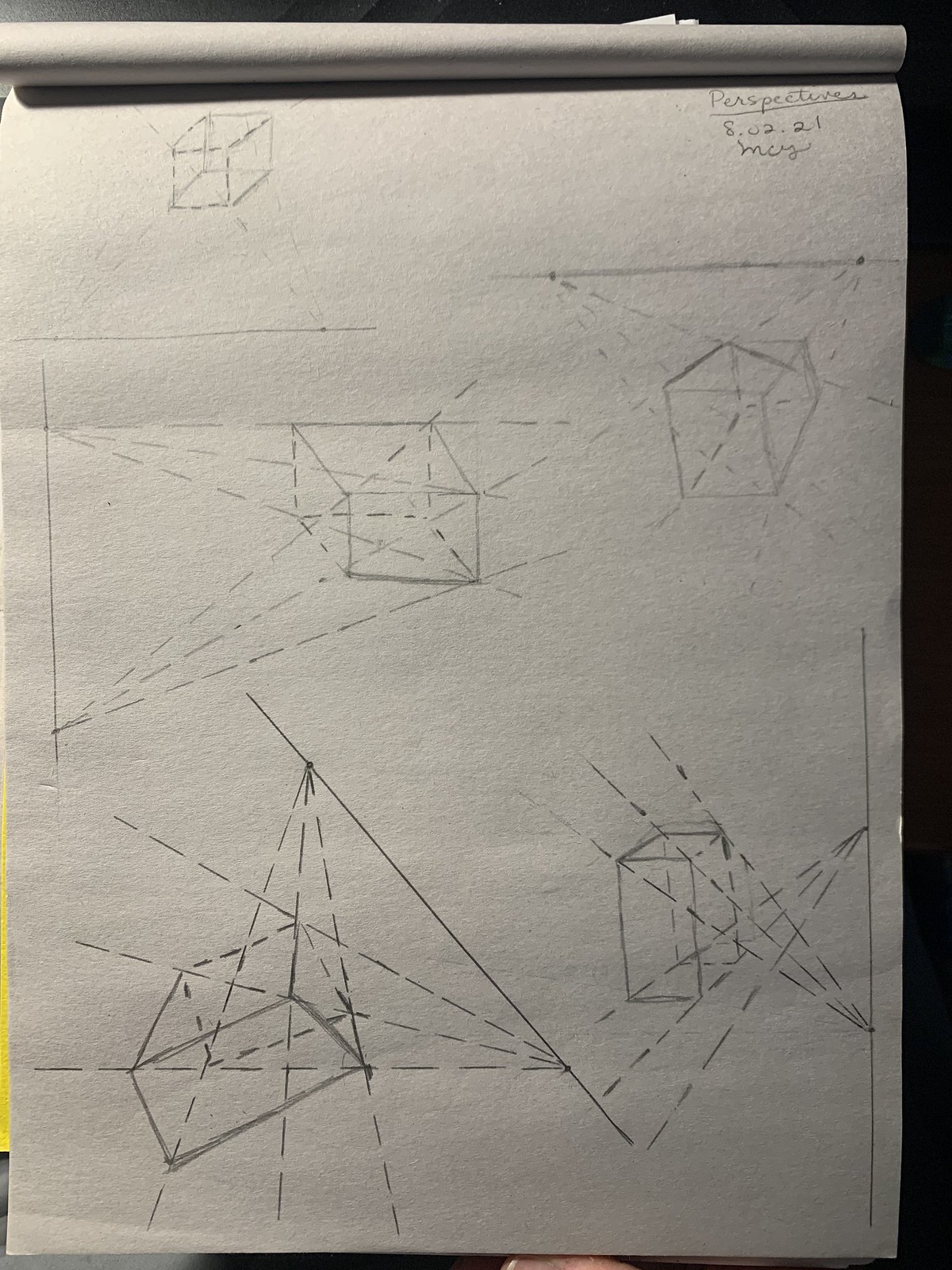An indoor photograph featuring a folded sheet of paper placed on a table. At the top right corner of the paper, the word "Perspectives" is elegantly written in cursive and underlined. Below this title, the date "8.02.21" is inscribed. Additionally, the name of the month appears in cursive writing. To the left of these inscriptions, there is a neatly drawn square box. Surrounding this box, various sketches of box-like shapes can be seen, each illustrated from different angles. Numerous arrows, pointing in multiple directions, are scattered across the sheet, adding a dynamic element to the otherwise orderly layout.